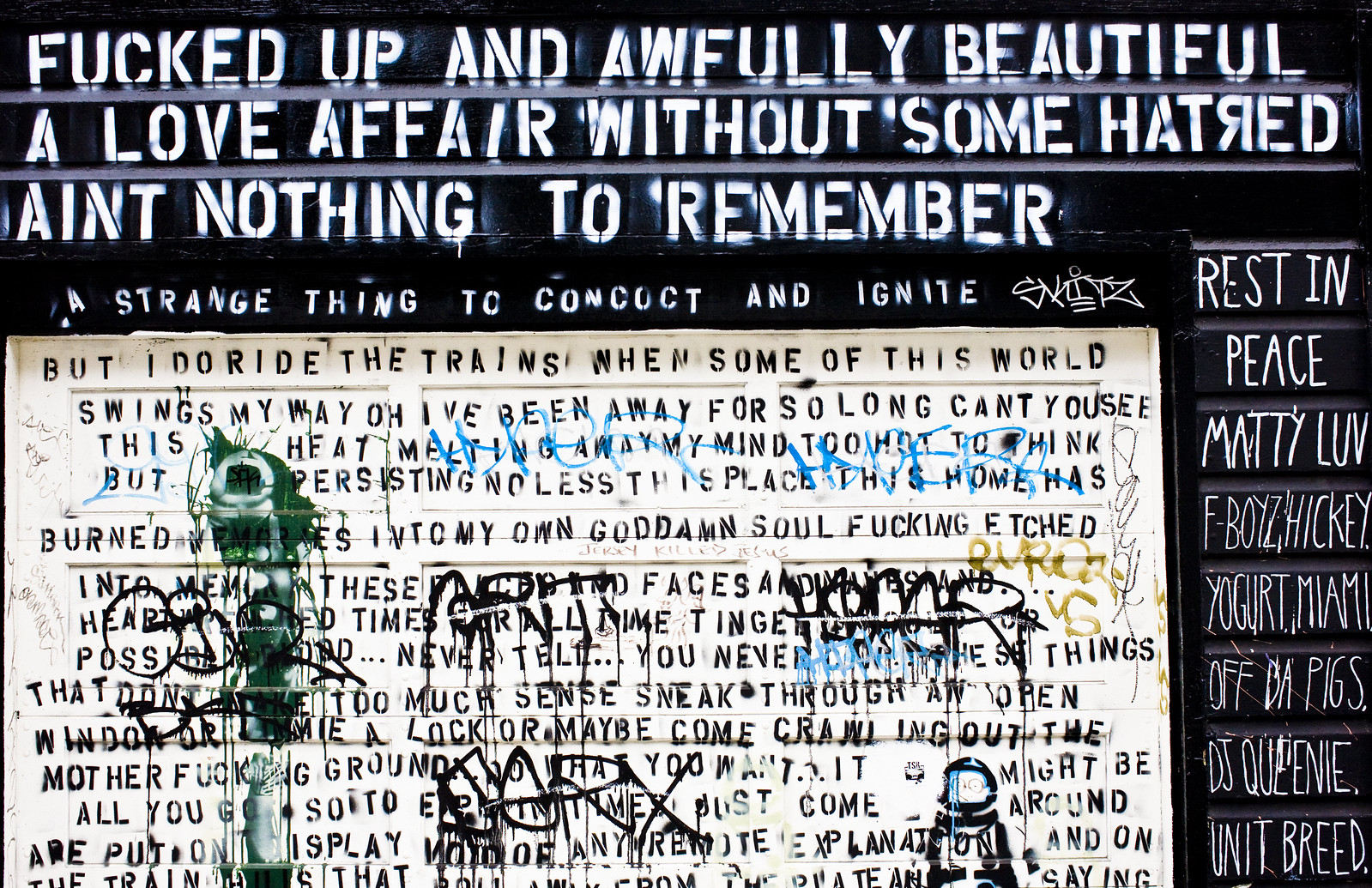The image presents a chaotic and intentionally messy black-and-white composition dominated by text and graffiti. At the top, large white capital letters boldly declare, "Fucked Up and Awfully Beautiful, A Love Affair Without Some Hatred and Nothing to Remember." Beneath this, in smaller white text, it reads, "A Strange Thing to Conduct and Ignite." The background predominantly black, contrasts with a white section below, enclosed in a box filled with an array of text and graffiti, including phrases like "Rest in Peace Maddie," "Love F Boys," "Hickey," "Yogurt," "Miami," and "Off the Pigs." This collage of disorderly black, green, blue, and gold scribbles evokes an intense, almost depressive atmosphere. The combination of poignant statements and random graffiti elements creates a visually striking and emotionally charged image.